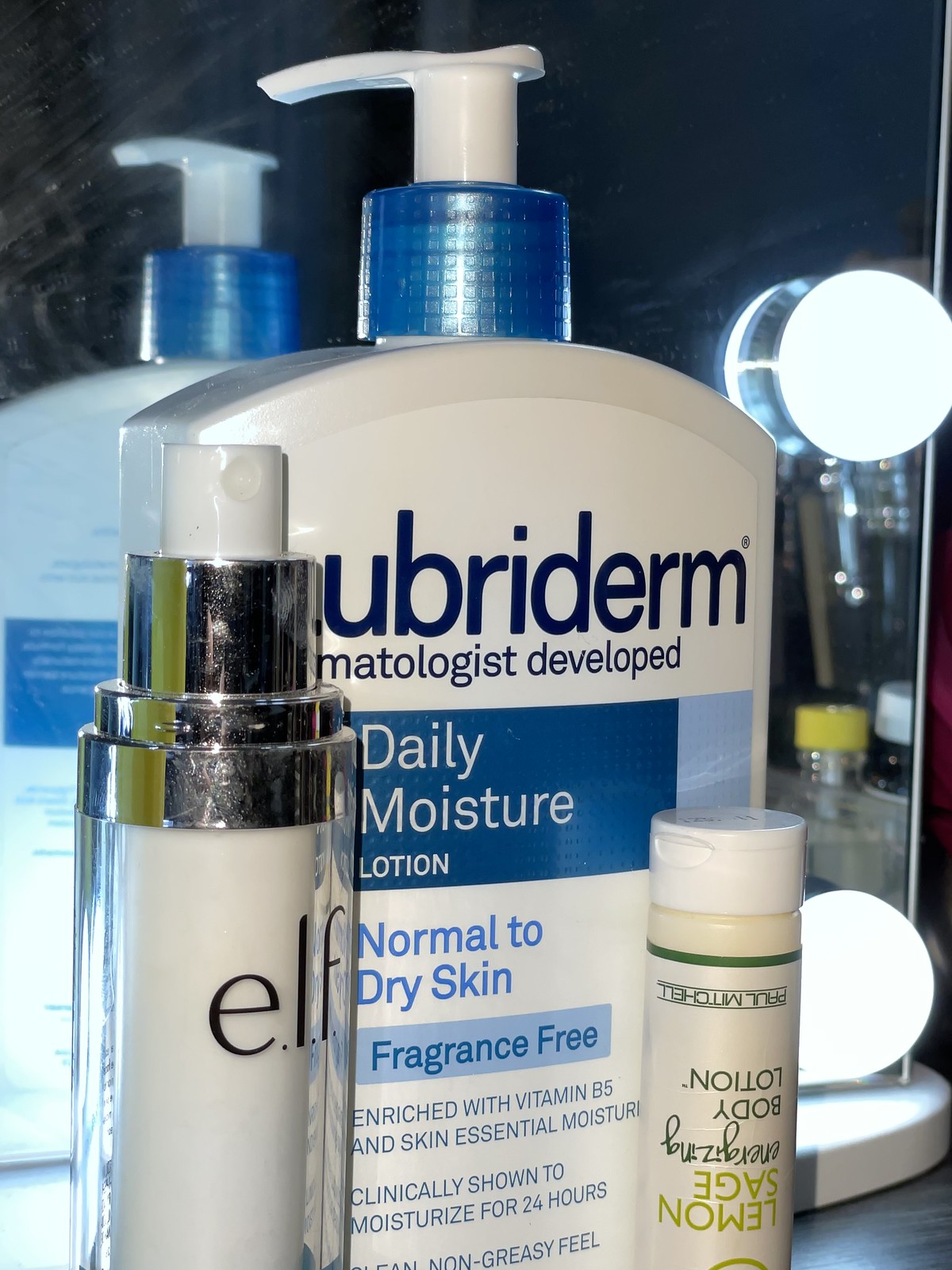A close-up photograph displays a bathroom shelf or counter adjacent to a sink, adorned with various skincare and hygiene products. Dominating the foreground is a large, white plastic bottle of Lubriderm dermatologist-developed daily moisture lotion, suitable for normal to dry skin. The bottle, characterized by its straight sides and rounded top, features a blue pump and cap. The Lubriderm logo is prominently printed in dark blue, while detailed product descriptions are written beneath: "Daily Moisture Lotion" in white, "Normal to Dry Skin" in medium blue, and a light blue banner declaring "Fragrance-Free, Enriched with Vitamin B5 and Skin-Essential Moisture." It highlights that the lotion is clinically shown to moisturize for 24 hours and has a non-greasy feel.

To the right of the Lubriderm bottle sits an upside-down, small sample-sized bottle of Paul Mitchell Lemon Sage Energizing Body Lotion. The clear bottle, from which its contents are visible, has a white cap situated at the top due to its inverted position. The labeling is notable for appearing upside-down while the bottle stands upright.

To the left of the Lubriderm is a larger, elegant glass bottle bearing the "ELF" label. It features a chrome top with a pump mechanism, encircled by a chrome ring and topped with a white pump. The bottle is filled with a white liquid that adds a sophisticated touch to the arrangement.

Adding depth to the scene, the back of the Lubriderm bottle is mirrored on the glossy, likely marble, black surface with white streaks at the left of the photo, suggesting an ambient low light setting. Contrasting the darker tones, the upper right corner showcases a lit round light fixture. Below this fixture, on a round stand, rests another white item beside a smaller bottle with a yellow cap, contributing to the orderly yet varied collection of bathroom essentials.